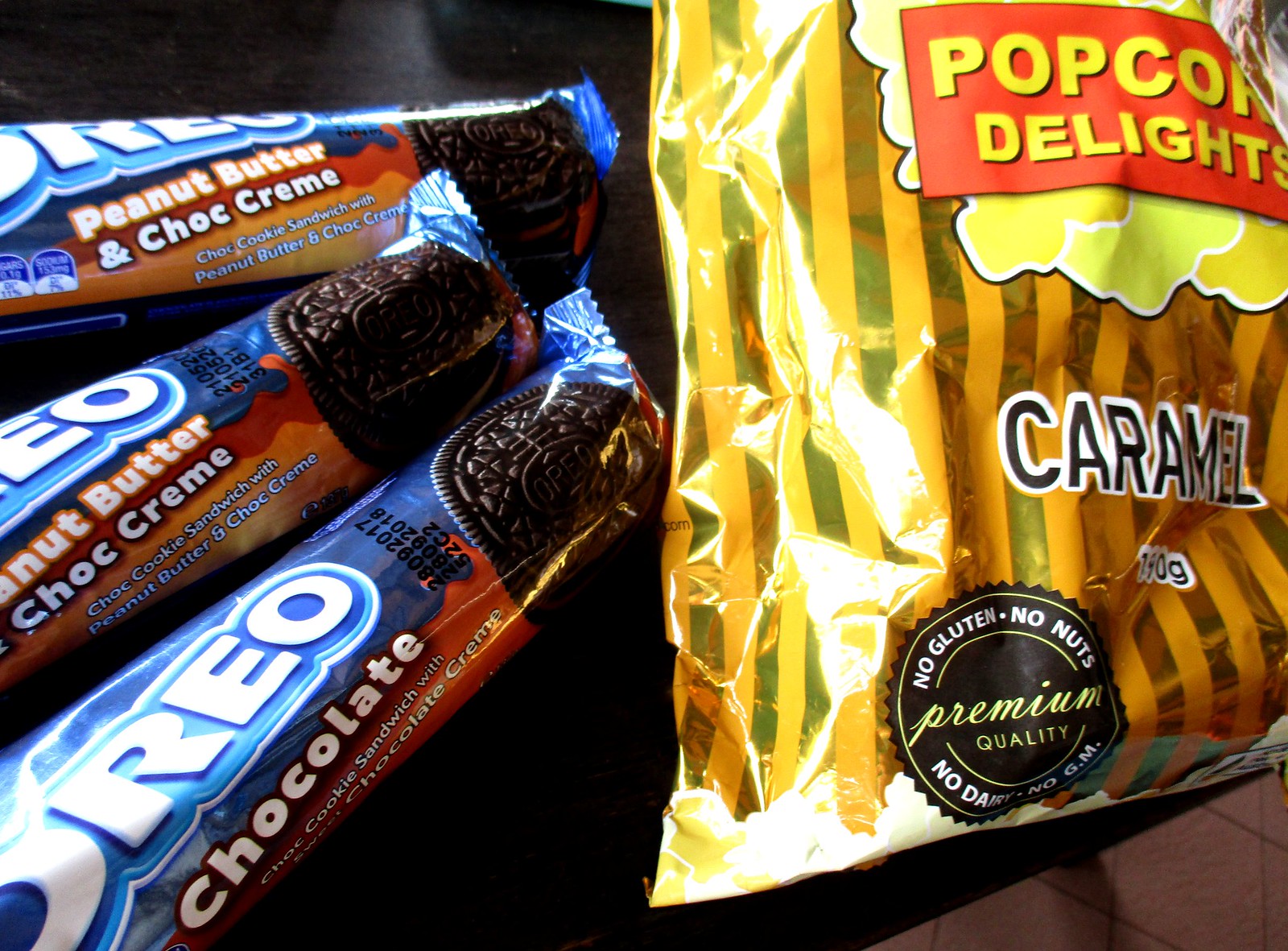This close-up photograph of snacks features a mix of Oreo cookies and caramel popcorn, branded as "Popcorn Delights." On the left, three packages of Oreos lie on their sides; the flavors include chocolate, peanut butter chocolate, and chocolate cream. Each package showcases the Oreo logo and images of the cookies, with color schemes of blue, white, black, and brown. To the right, a vertically positioned bag of caramel popcorn is displayed, adorned with gold and red stripes and the text "Caramel, Premium Quality." The "Popcorn Delights" branding and a stylized drawing of popcorn are visible on the bag. The entire arrangement rests on what appears to be a kitchen table, illuminated by indoor artificial lighting. The popcorn bag's colors are predominantly golden yellow and gold, while the Oreo packaging predominantly features blue tones with red accents.